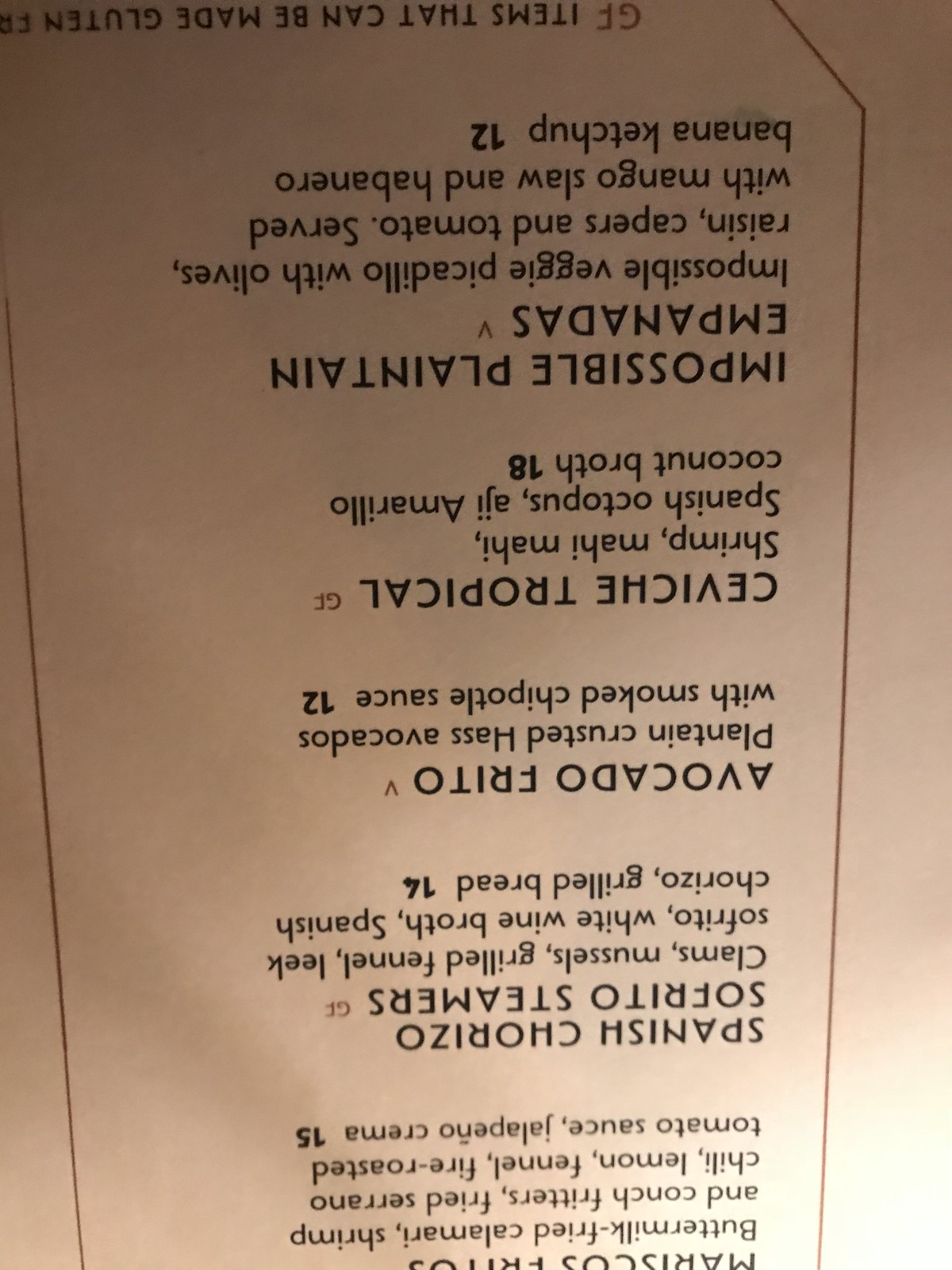This image captures a photograph of an off-white menu with very clear black font. The menu is displayed upside down on the screen. At the top of the menu (which appears at the bottom of the picture due to the upside-down orientation), there is a slightly cut-off heading that appears to read "Moriscos Fritos." Below this heading, the first detailed menu item is "Buttermilk Fried Calamari, Shrimp and Conch Fritters," which includes fried Serrano chili, lemon, fennel, fire-roasted tomato sauce, and jalapeño crema, priced at $15.

Following this, the next item listed is "Spanish Chorizo Sofrito Steamers," which consists of clams, mussels, grilled fennel, leek, sofrito, white wine broth, and Spanish chorizo grilled bread, priced at $14.

The third item is "Avocado Frito" marked with a "V" indicating it is a vegan option. This dish features plantain-crusted Haas avocados with smoked chipotle sauce and is priced at $12.

Next, the menu lists "Ceviche Tropical," which includes shrimp, mahi-mahi, Spanish octopus, ají amarillo, and coconut broth, priced at $18.

At the bottom of the menu (or the top of the picture), there is "Impossible Plantain Empanadas," another vegan option. This dish contains Impossible veggie picadillo with olives, raisins, capers, and tomatoes, served with mango slaw and habanero banana ketchup, priced at $12.

Additionally, there is a note indicating "GF" for gluten-free items that can be made with gluten.